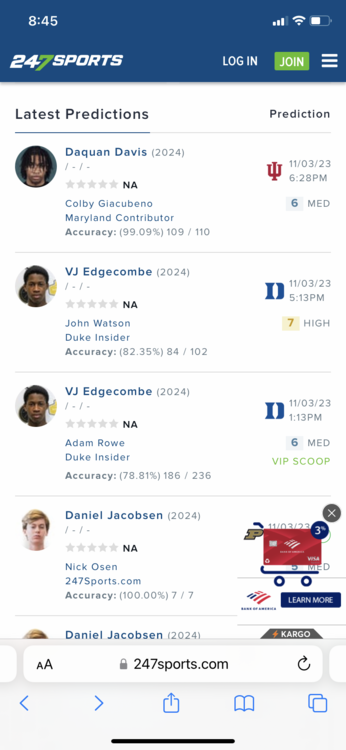The screenshot captures a moment on a sports prediction website, accessed via a smartphone at 8:45. The device displays three cellular service bars, full-strength Wi-Fi, and approximately half of its battery capacity. At the top of the website, options for logging in, joining, and a three-line hamburger drop-down menu are visible. The page prominently features the "Latest Predictions" section.

Highlighted first is Daquan Davis, a 2024 prospect with no star rating, followed by Colby Ghiabarno, a Maryland contributor with an impressive prediction accuracy of 99.9% based on 109 correct predictions out of 110. 

Next, Vijay Edgecombe, another 2024 prospect, also displays no star rating. John Watson, a Duke insider, showcases an accuracy of 82.35%, having made 84 correct predictions out of 102 attempts. Vijay Edgecombe appears again, still without a star rating, and Adam Rowe, another Duke insider, exhibits an accuracy of 78.81%, with 186 correct predictions out of 236.

Finally, Daniel Jacobson, similarly listed without stars, is accompanied by Nick Olson from 24-7 Sports. Nick boasts a perfect accuracy of 100%, successfully navigating 7 predictions out of 7 attempts.